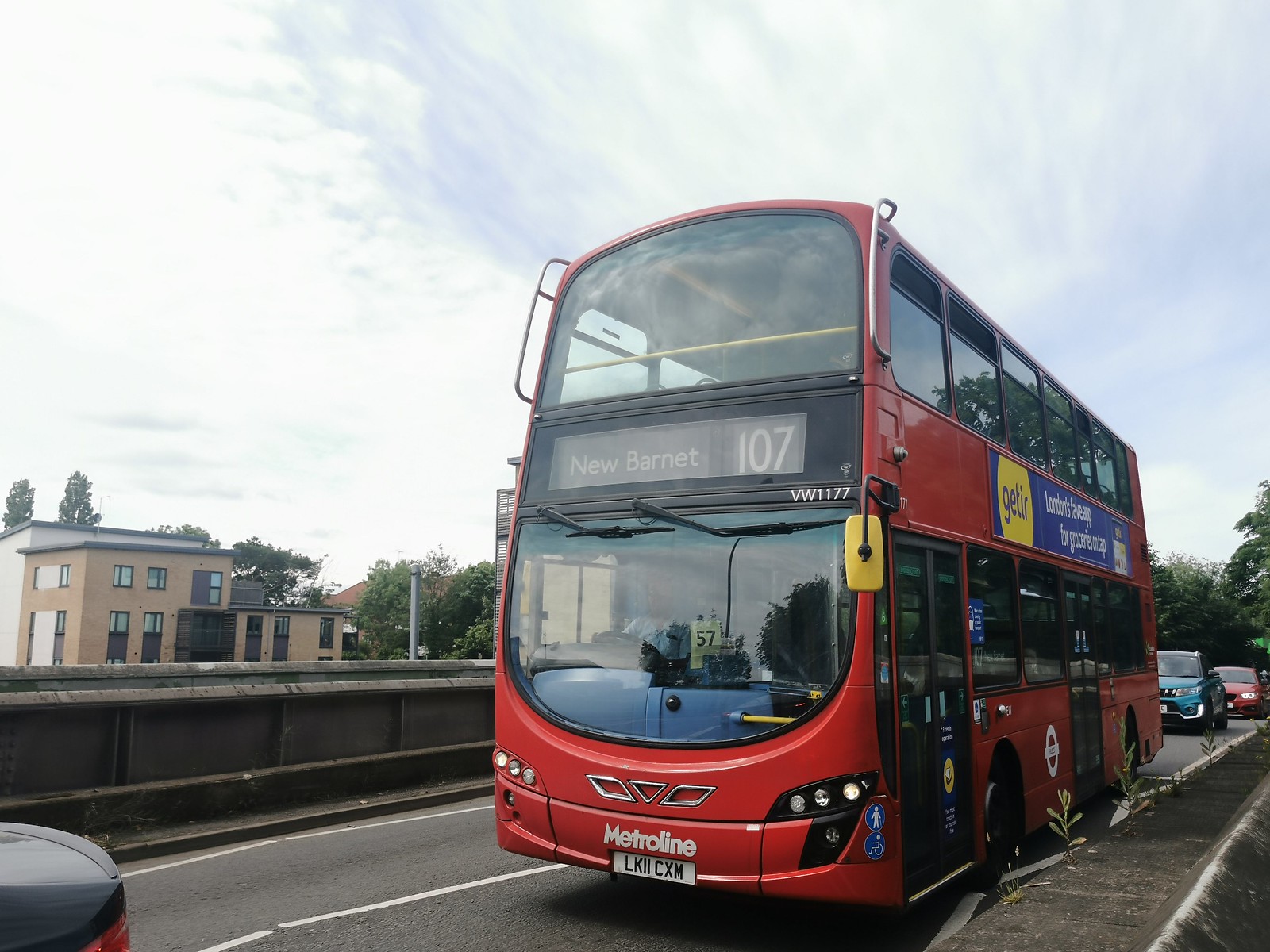The image depicts a red double-decker Metroline bus, prominently featuring the route number "107" to New Barnet on the front above a large windshield, with "Metroline" inscribed beneath it. The bus, which carries the license plate "LK11 CXM," is traveling down a city street during the daytime, with streaked clouds visible in the sky. There are multiple buildings, possibly storefronts, in the background along with a road divider. The bus advertising, a blue banner with yellow elements, promotes an app, although some text is obscured. You can also see the bus has two doors, one at the front and another in the middle. Behind the bus, a blue car and a red car are visible, while trees can be seen in the distance. The scene suggests a busy urban environment.